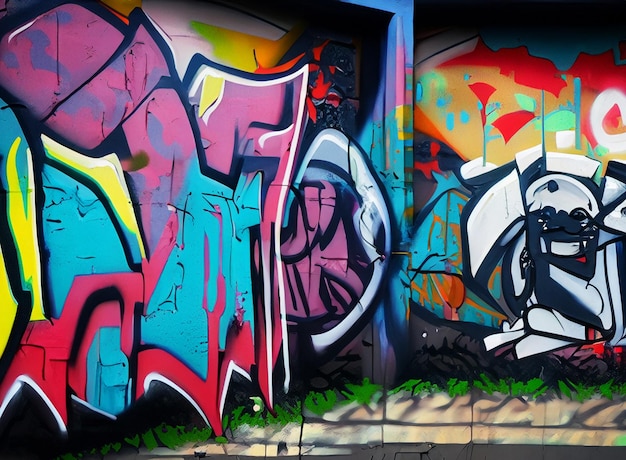The image showcases modern graffiti street art, rich in vivid and saturated colors like blues, reds, purples, yellows, and whites. It stretches across the wall from left to right, creating an intricate and almost chaotic mosaic. On the right-hand side, reds, greens, and yellows dominate, forming various shapes and sizes. Among these colorful patterns, a white face with expressive eyes and a black face with teeth showing can be discerned, possibly with a body below and legs crossed.

At the bottom of the image, green paint suggests grass, revealing glimpses of the beige wall beneath, indicating layers of paint built up over time. The graffiti appears to be an amalgamation of multiple artists' works, overlapping to the point where individual pieces are indistinguishable, creating an abstract visual experience. There's also an impression of a purple-faced figure wearing a hood on the left side, and above it, some kind of creature. The overall composition is bold, with the saturated colors forming a near-indiscernible collage of shapes and patterns. While the wall and possible architectural elements can be faintly seen beneath, the true depth of the artwork remains open to interpretation.